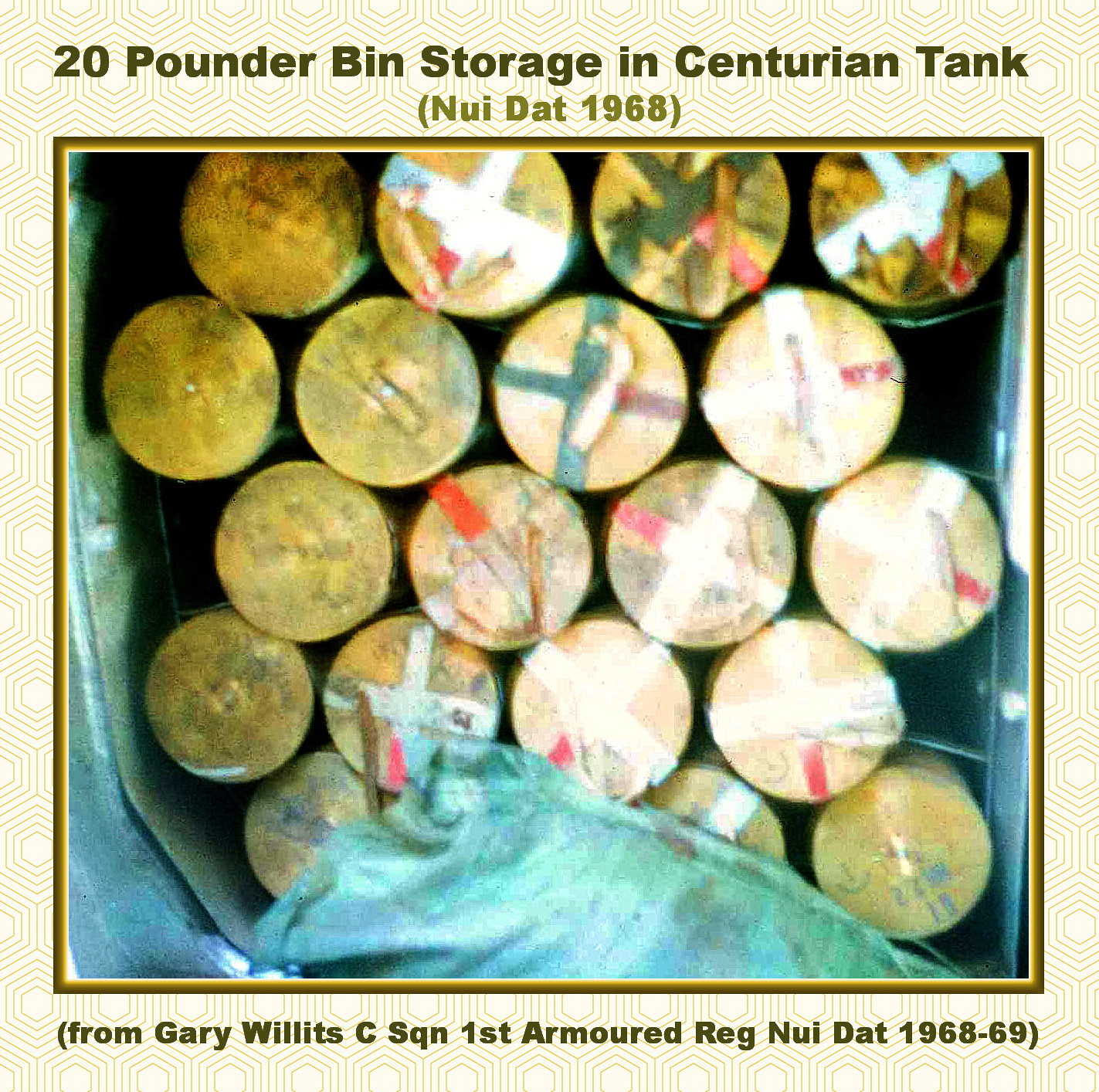The photograph is a colored image, framed with a designed border that varies in description, either pink or greenish-brown. The frame encloses a collection of circular objects, some appearing in brown, dirty yellow-green, and others in pink or peach. Several of these circles are marked with colored X's. Captioned in black at the top is the text "20 Pounder Bin Storage in Centurion Tank, Nui Dot 1968 (Nguoi Dot 1968)," suggesting a Vietnamese context. Below the image, it reads, "From Gary Willett's C-Squadron, First Armored Regiment, Nui Dot 1968-1969."